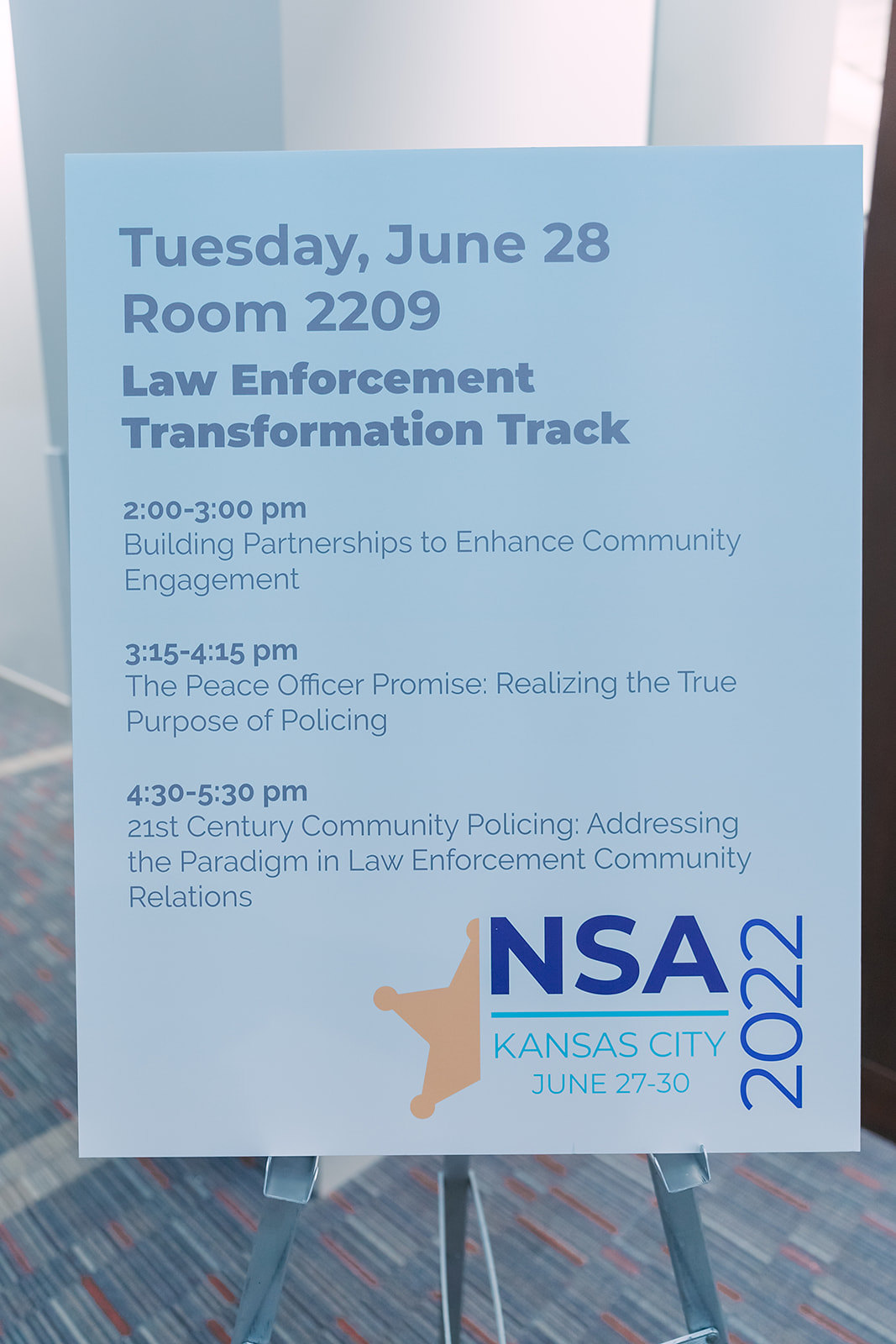The image features a poster mounted on a metal support stand, placed on blue, orange, and white carpeting. The poster has a gradient blue background, transitioning from darker at the top to lighter at the bottom. It features dark blue lettering, making the text easily readable. The poster details an event schedule for Tuesday, June 28th, in Room 2209 under the "Law Enforcement Transformation Track". The schedule includes: "2 to 3 p.m. - Building Partnerships to Enhance Community Engagement", "3.15 to 4.15 p.m. - The Peace Officer Promise, Realizing the True Purpose of Policing", and "4.30 to 5.30 p.m. - 21st Century Community Policing, Addressing the Paradigm in Law Enforcement Community Relations". At the bottom of the poster, there is an orange or red half-badge design along with "NSA Kansas City, June 27-30, 2022".